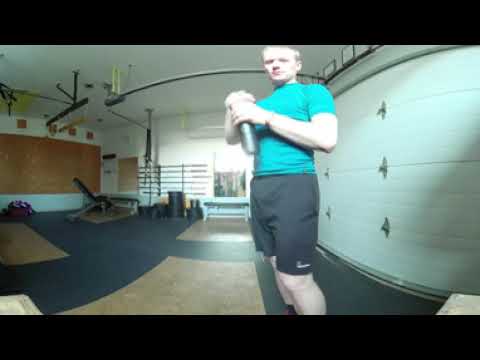In the photograph, a fit, blonde-haired white man stands facing the viewer inside a spacious, dimly lit home gym, likely situated in a garage. He wears a turquoise short-sleeved shirt and black workout shorts featuring a white Nike logo near the left knee. He holds a gray cylindrical object, possibly a water bottle, with his right hand gripping the top and his left arm resting across his chest. The gym's floor comprises black and tan mats arranged in a pattern, and various pieces of exercise equipment, including a weight bench with black weights, populate the background. Behind him, a white garage door is visible on the right, complete with its mechanism extending across the ceiling, and the room features a mix of white walls, some with brown accents, and black ceiling fixtures. The overall atmosphere is that of an athletic, well-equipped indoor space, albeit with slightly distorted perspective due to the photograph's lens.